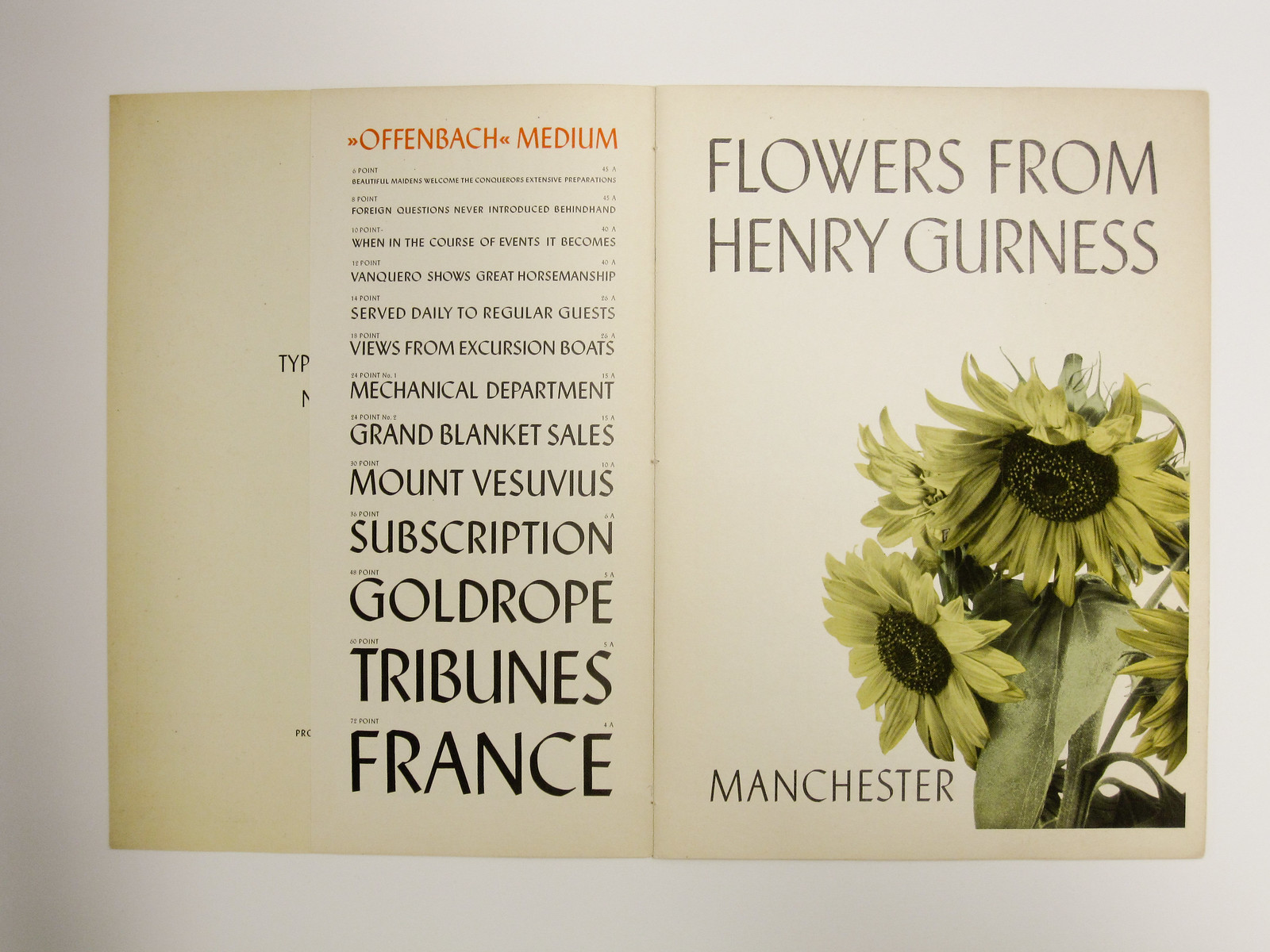The image features an open book or sheet of paper placed on a white background. On the right page, there is a photograph of yellow sunflowers that appear to be wilting. Above the photograph, the text reads "Flowers from Henry Guerness," and below it, "Manchester." 

On the left page, the top text "Offenbach Medium" is written in orange font. Below that, in black text of varying and progressively increasing sizes, are phrases such as: "From beautiful Noreen's welcome to consequences extensive preparations," "When in the course of events it becomes," "Vaccaro shows great horsemanship," "Served daily to regular guests," "Views from excursion boats," "Mechanical department," "Grand blanket sales," "Mount Vesuvius," "Subscription," "Gold rope," "Tribune," and "France." The font sizes for these phrases increase from 5 point to 72 point as they descend down the page. The primary colors in the photograph are white, black, orange, and yellow.